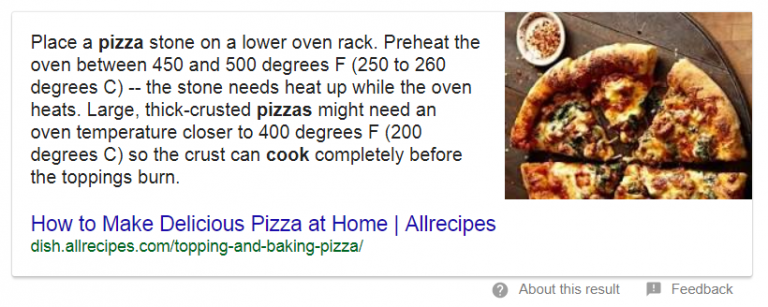This image captures a beautifully baked cheese pizza resting on a pizza stone. The pizza, with its thick, golden-brown crust reminiscent of a deep-dish style, is generously topped with melted cheese and savory Italian sausage, complemented by fresh spinach. Rustic and appetizing, the pizza sits invitingly on the stone rack, highlighting the artisanal touch of being stone-baked. Adjacent to the pizza are crushed red pepper flakes in a small condiment cup, adding a touch of spice for those who desire it. 

This snapshot is sourced from a recipe page on AllRecipes.com, detailing how to create a delicious homemade pizza. According to the instructions, place the pizza stone on a lower rack of your oven and preheat the oven to a temperature between 450 and 500 degrees Fahrenheit. The stone must be heated concurrently with the oven. For large, thick-crusted pizzas, adjust the oven temperature to approximately 400 degrees Fahrenheit to ensure the crust is fully cooked without overcooking the toppings.